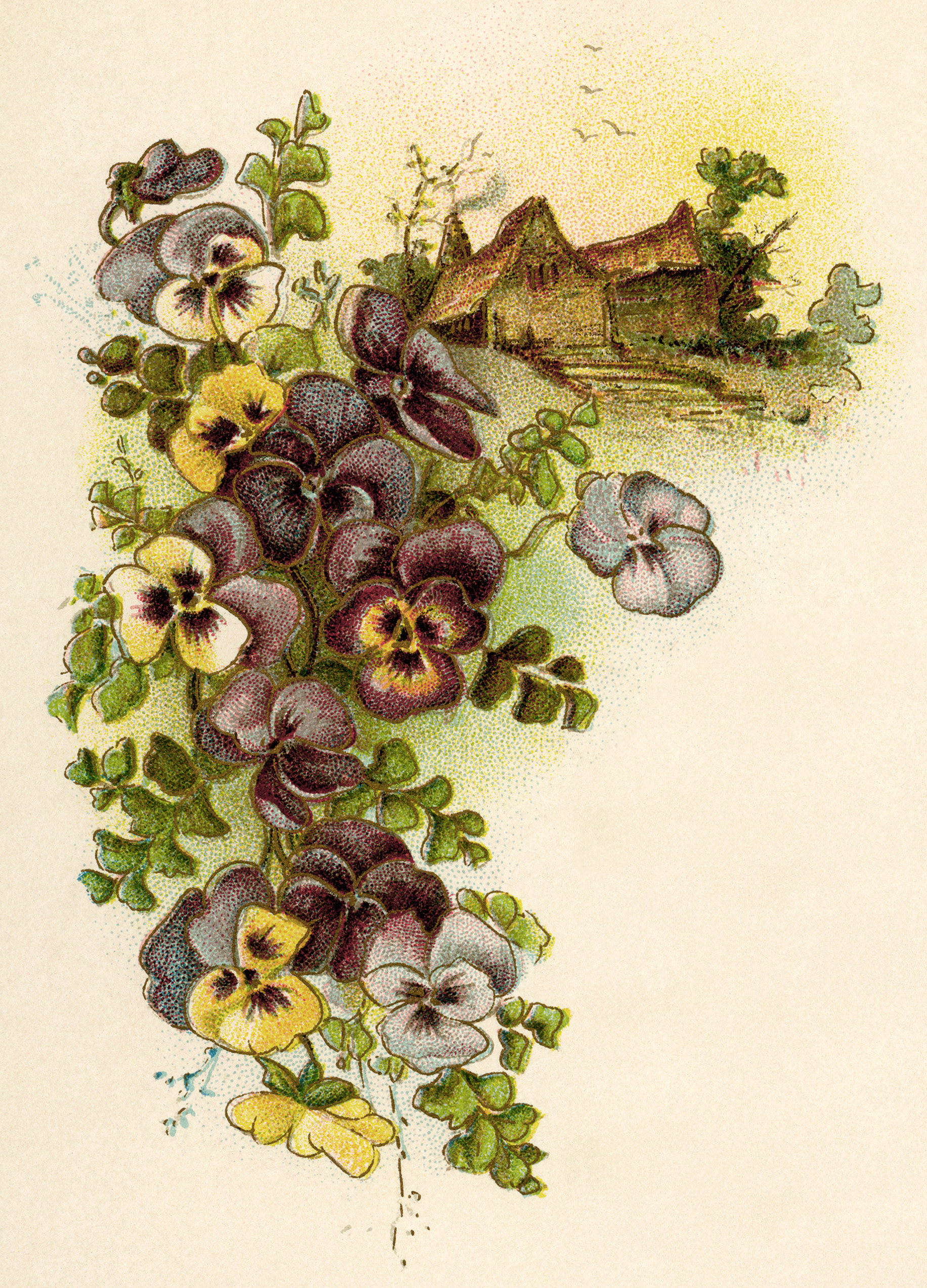The image is a beautifully detailed illustration against a tan, aged-looking background, reminiscent of vintage artwork. On the left side, a cascading vine is adorned with vibrant pansy flowers in shades of yellow, purple, dark purple, and white. Each flower features intricate details, with petals varying from yellow to purple and white, and delicate leaves surrounding them. The flowers and vines create a flowing, vertical arrangement from top to bottom.

In the background, nestled amidst lush green trees, are two old, worn-down wooden cabins. One cabin, positioned slightly above the other, lies on a hill with a visible pathway leading down. Both cabins have triangle-shaped roofs, contributing a rustic charm to the scene. Above the cabins, small birds are seen flying, adding a serene touch. The illustration is laid on top of a tan fabric or canvas, enhancing its timeless and peaceful aura.